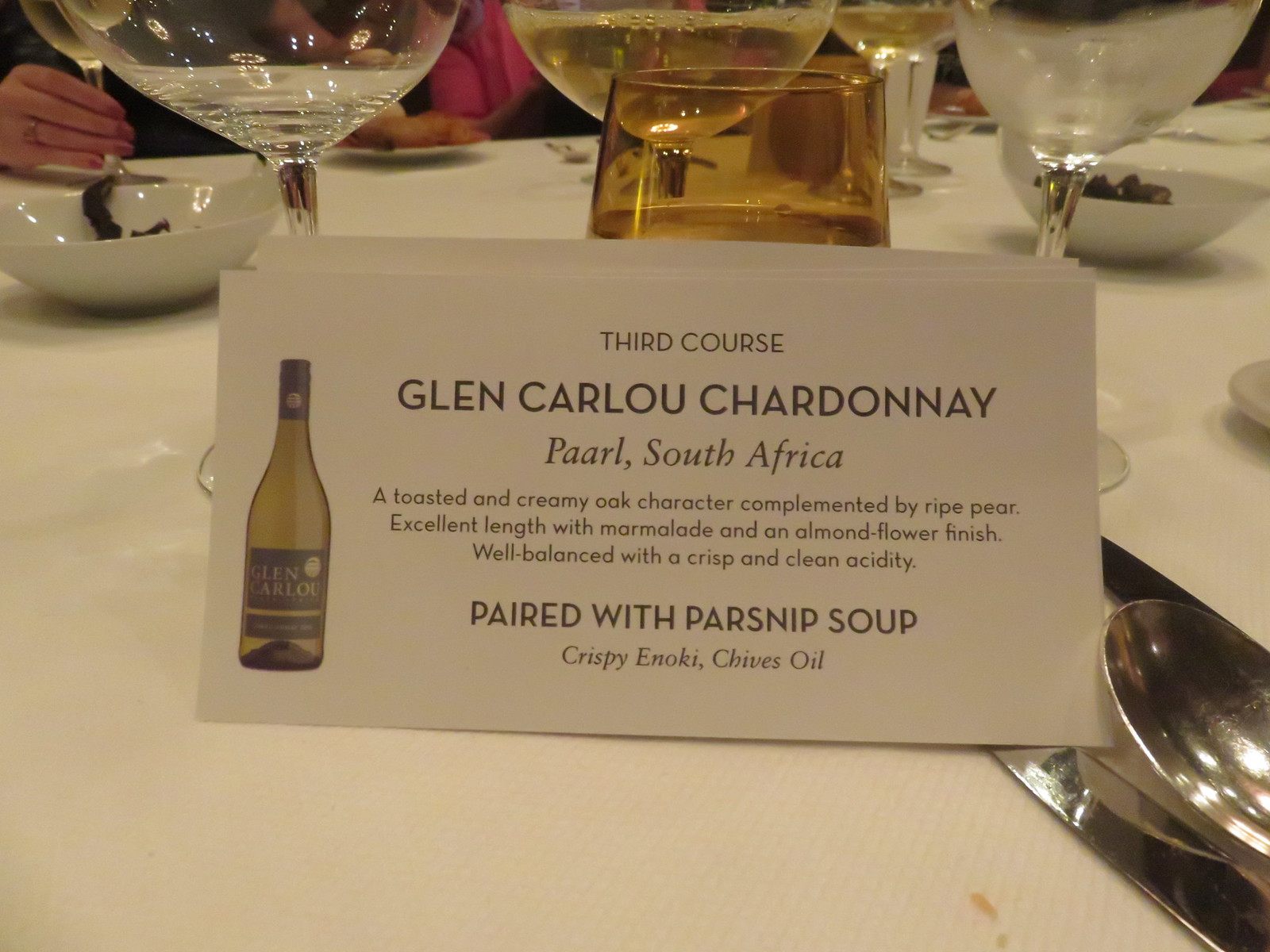The photograph captures a meticulously set dinner table dressed with a white cloth. At the center of the image is a pristine white place card, propped up against the stem of a wine glass. This card features a detailed description of a wine, specifically a Glen Carlou Chardonnay from Paarl, South Africa, paired with a third course. Surrounding it are three wine glasses arranged at the top, each holding different liquids: one with white wine, another with a yellowish hue, and the third filled with clear water. To the right of the scene, shiny silverware, including a spoon, adds a polished touch. The card itself, surrounded by additional dining items like dishes and cutlery, showcases an image of a Chardonnay bottle and provides an eloquent wine description, highlighting its toasted and creamy oak character, ripe pear notes, and a well-balanced finish with marmalade and almond flower nuances. It suggests pairing this wine with parsnip soup garnished with crispy enoki, chives, and oil, emphasizing an excellent length and crisp, clean acidity. The colors prominent in the image include whites, greens, oranges, grays, and purples.